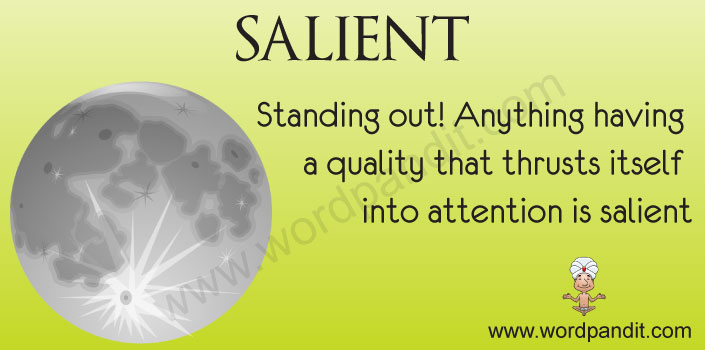The image features a gradient green background that transitions from a darker shade at the bottom to a lighter, dull lime green at the top. On the left-hand side, there is a digital image of the moon with dark spots and a bright light at its base. At the top of the image, the title "SALIENT" is prominently displayed in black, uppercase text. Below this, the definition reads, "Standing out. Anything having a quality that thrusts itself into attention is salient." On the bottom right-hand corner, a digital figure, resembling a genie or guru, sits in a lotus position wearing a white turban. Below this figure, the URL "www.wordpandit.com" is displayed. Additionally, the website address "www.wordpandit.com" appears in greyed-out text, overlaying the entire image as a watermark. The combination of the vibrant background, striking moon imagery, and clear educational content makes the image visually appealing and informative.